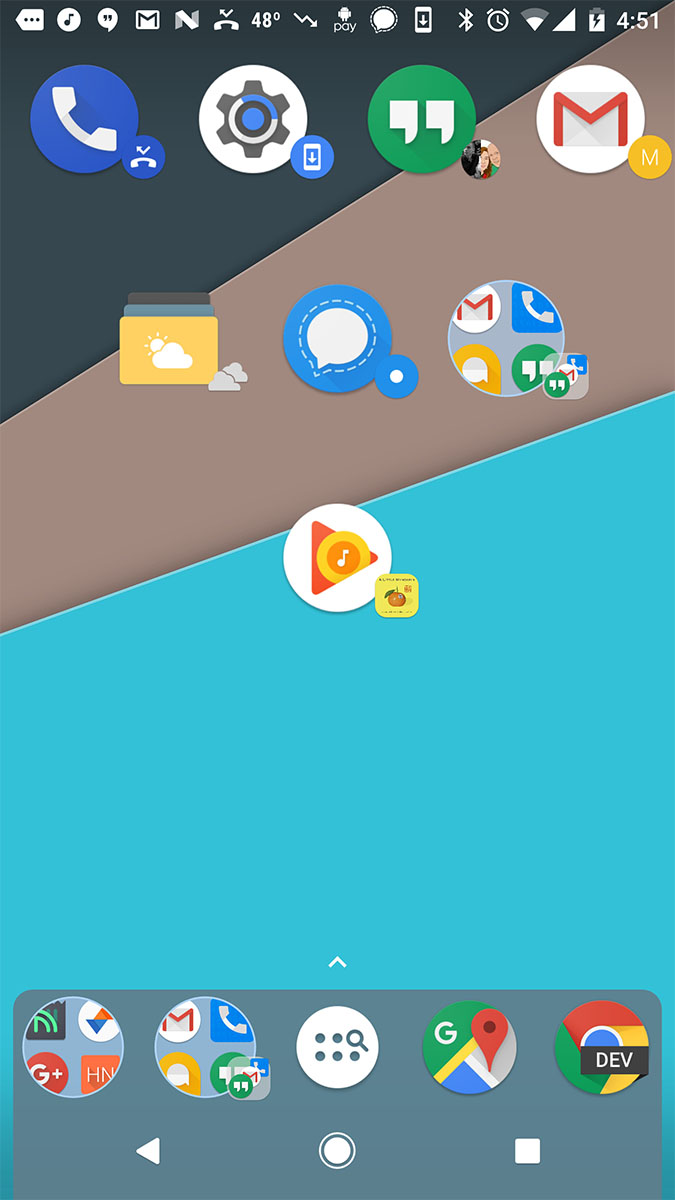This is a detailed caption for an image of a phone screenshot in portrait orientation, approximately two to three times taller than it is wide. The phone's background features diagonal lines descending from the top right to the bottom left, dividing the screen into three color sections: a dark bluish-black, a grayish-brown, and a light blue, with the light blue occupying the majority of the screen.

At the top of the screen, a horizontal row of icons is visible, which includes:
- An arrow with three dots pointing left
- A circle with a musical note inside
- A text bubble
- The Google Mail icon
- A grayed-out or blurry "N"
- A missed call notification
- A temperature reading of 48 degrees
- A downward pointing arrow
- The Android Pay app
- A white bubble
- A download symbol
- A Bluetooth icon
- An alarm clock icon
- A Wi-Fi meter at about half strength
- A network service meter showing full signal
- A vertical battery icon fully charged with a white meter
- A charging icon featuring a lightning bolt
- The current time displayed as 4:51

Below these icons, there is another set of circular icons representing various apps, including but not limited to phone, settings, chat, email, and other unfamiliar icons. More icons are placed at the bottom of the screen, though their specifics are not detailed.